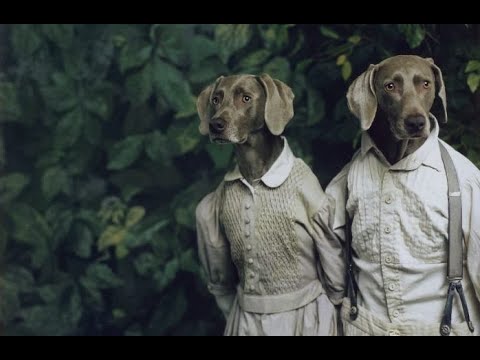This image depicts a surreal, realistic photograph of two black Labrador dogs with human bodies, dressed in formal attire. Both dogs stand upright in front of a leafy background, their canine heads and expressive faces exhibiting a melancholic demeanor. The body of the male dog is attired in a white dress shirt with grey suspenders, while the female dog wears a white button-down blouse and dress. The human forms possess human arms, waists, and chests, but their heads are unmistakably those of dogs, complete with grey ears, black noses, and downcast eyes. Behind them, the scene is filled with a lush array of green leaves and trees, with subtle shadows adding depth to the forest-like setting. The dogs' paws appear to be hidden behind their backs, adding to the odd human-like posture they maintain while gazing slightly apart into the distance.